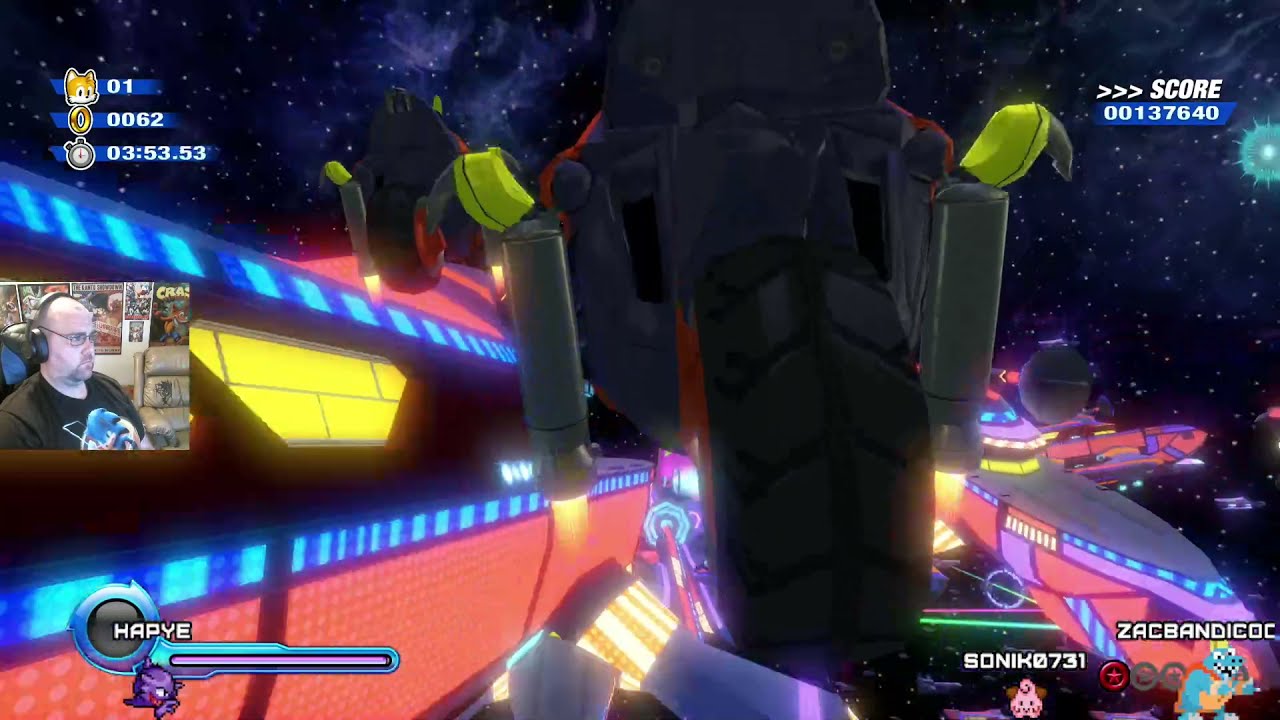This image is a detailed screenshot or possibly a live stream of a space-themed video game. The focal point features a male streamer inset on the left side, appearing intently engaged in gameplay. He is a bald Caucasian man wearing glasses, a headset, and a distinctive black Sonic the Hedgehog t-shirt. Behind him, posters adorn the wall. 

The game's visual presents a dark outer space background, peppered with oscillating white dots, reminiscent of stars. The scene is dominated by colorful spaceships with blue and red lighting accents, forming a jumbled cluster. A flying motorcycle, viewed primarily from the back wheel, seems to be navigating through this vibrant space.

The game's HUD (Heads-Up Display) provides additional context. In the upper left corner, there's an indication of a Sonic-related element, showing Tails with one life left, 62 gold rings collected, and a timer displaying 3 minutes and 53 seconds. The scoreboard in the top right corner reads 00137640. At the bottom right, usernames like Sonicle731 and Zap Bandicock (likely intended to be Zap Bandicoot) are visible. A status bar in the lower left with the label "HAPYE" rounds out the display elements.